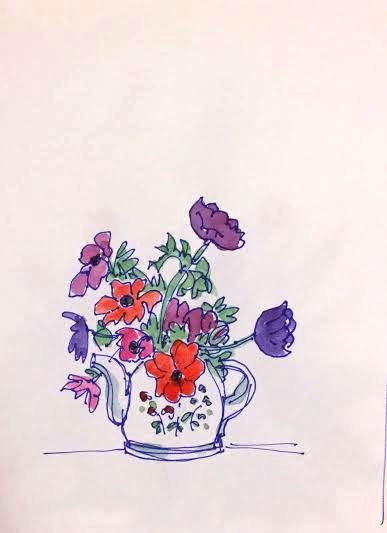A vibrant painting showcases a collection of multi-colored flowers arranged in a white vase or teapot. The floral assortment includes two purple flowers, three maroon, two pink, two orange, and one dark pink blossom. All flowers are surrounded by lush green leaves. The center of four of these flowers are marked by distinctive black circles. The white teapot itself is adorned with small red flowers accompanied by green leaves, and delicate blue butterflies, adding an extra layer of charm to the composition. The entire scene is set against a plain white background, with a line running under the teapot, grounding the arrangement and adding depth to the display.